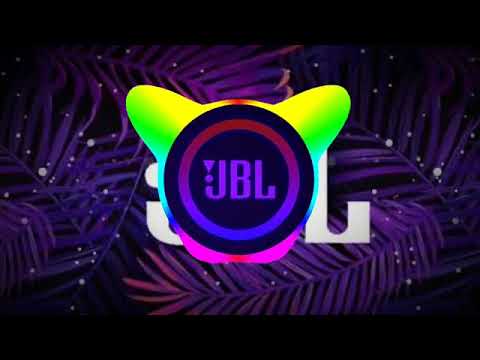In the center of the image, the prominent text "JBL" is displayed in purple letters. Surrounding the "JBL" are circles with multi-colored hues of purple and blue, while the background within these circles is a darker shade of purple compared to the font. Adding structure to the design, there's a border of dark purple. Another key feature is an abstract drawing that resembles a cat with lime green and yellow cat ears overlaying the text, partially obscuring the "JBL" so that only the ends of the 'J' and 'L' are visible.

The artistic composition contains a dark, starry night sky with white dots, serving as the backdrop. Throughout the image, purple leaves akin to marijuana or fern leaves appear, displaying shades ranging from reddish-purple to bluish-purple. The bottom and top edges of the image are marked by black bars devoid of any patterns or dots. The overall theme of the image suggests an outer space scenery merged with vibrant, digital artwork, creating a bright yet dark and mysterious ambiance. There is no depiction of any humans in the image, solely focusing on the logo and abstract elements.